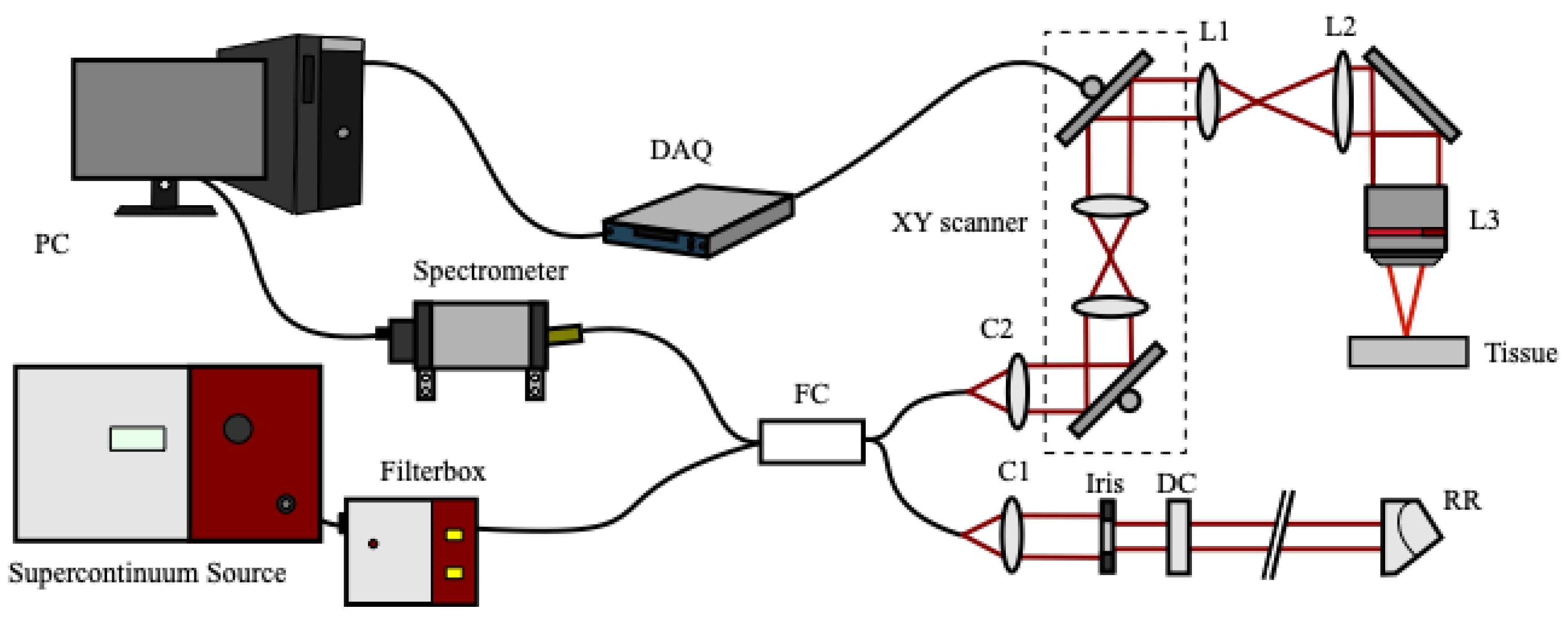The image depicts a detailed and technical diagram with a white background illustrating the interconnected system of scientific equipment. The diagram begins at the upper left with a black PC tower and monitor with a gray screen. The PC is connected via various wires to multiple devices including a DAQ (Data Acquisition Device) and a spectrometer. A cord from the DAQ extends to an XY scanner, which connects sequentially to labeled components L1, L2, and L3, before reaching a section marked "tissue.”

In the bottom left, another component labeled "super continuum source" is linked to a "filter box" through black lines. This filter box is subsequently connected to a device labeled FC, which then connects to further components C1, C2, Iris, DC, and RR. The diagram uses color coding with lines and boxes in shades of gray, black, and red to illustrate the flow and connections between the various elements. The labels and arrows aim to demonstrate the setup for a scientific or computational process, requiring specialized knowledge to fully comprehend.